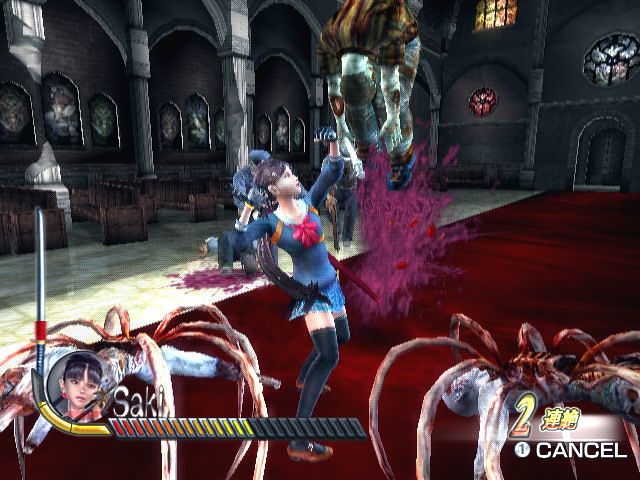In a suspenseful scene from a video game, the character Saki takes center stage, clad in a striking blue outfit adorned with a pink bow at the center. Saki, an Asian warrior with flowing black hair, confronts a formidable array of very large spiders. Adding to the chaos, another enemy descends menacingly from the ceiling. Saki's attire further includes thigh-high tights and red shoes, emphasizing her vibrant and dynamic appearance. The battle unfolds within the ornate confines of a church, amplifying the tension and drama. Positioned on the side is a distinctive sword, featuring a red band near the bottom and a blue handle, poised for action. A user interface is visible at the bottom of the screen, displaying options that include "Two" and "Cancel," indicative of the strategic choices available to the player controlling Saki. The detailed setting, combined with Saki's courageous stance, captures a pivotal moment of combat and strategy in this enthralling video game environment.